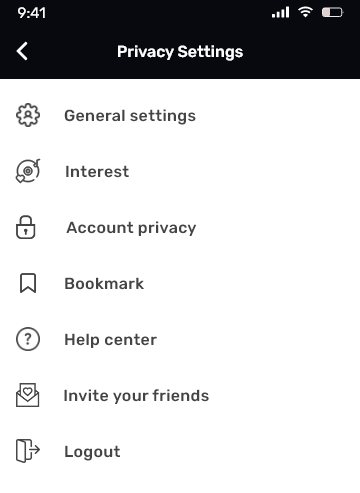The image is a screenshot from a mobile app, captured at 9:41 AM, as indicated by the time displayed at the top. The device shows full cell signal, connected to Wi-Fi, and the battery is approximately one-third charged. Below the status bar, the header titled "Privacy Settings" is displayed in white font on a black background. 

The main content of the screenshot features a section with a white background and black text, listing various settings options:

1. **General Settings**: Not specifically iconized.
2. **Interests**: Represented by a gear with a cartoon figure from the shoulders up, depicted as a circle on top of a downward-facing parenthesis.
3. **Account Privacy**: Denoted by a padlock icon.
4. **Bookmark**: Illustrated with a ribbon icon featuring an open chevron at the bottom.
5. **Help Center**: Symbolized by a circle containing a question mark.
6. **Invite Your Friends**: Indicated by an envelope with a letter inside, marked with a heart.
7. **Log Out**: Represented by an open door with an arrow pointing to the right.

The layout is clear, with recognizable icons accompanying each option, designed to help users easily navigate through their account settings.